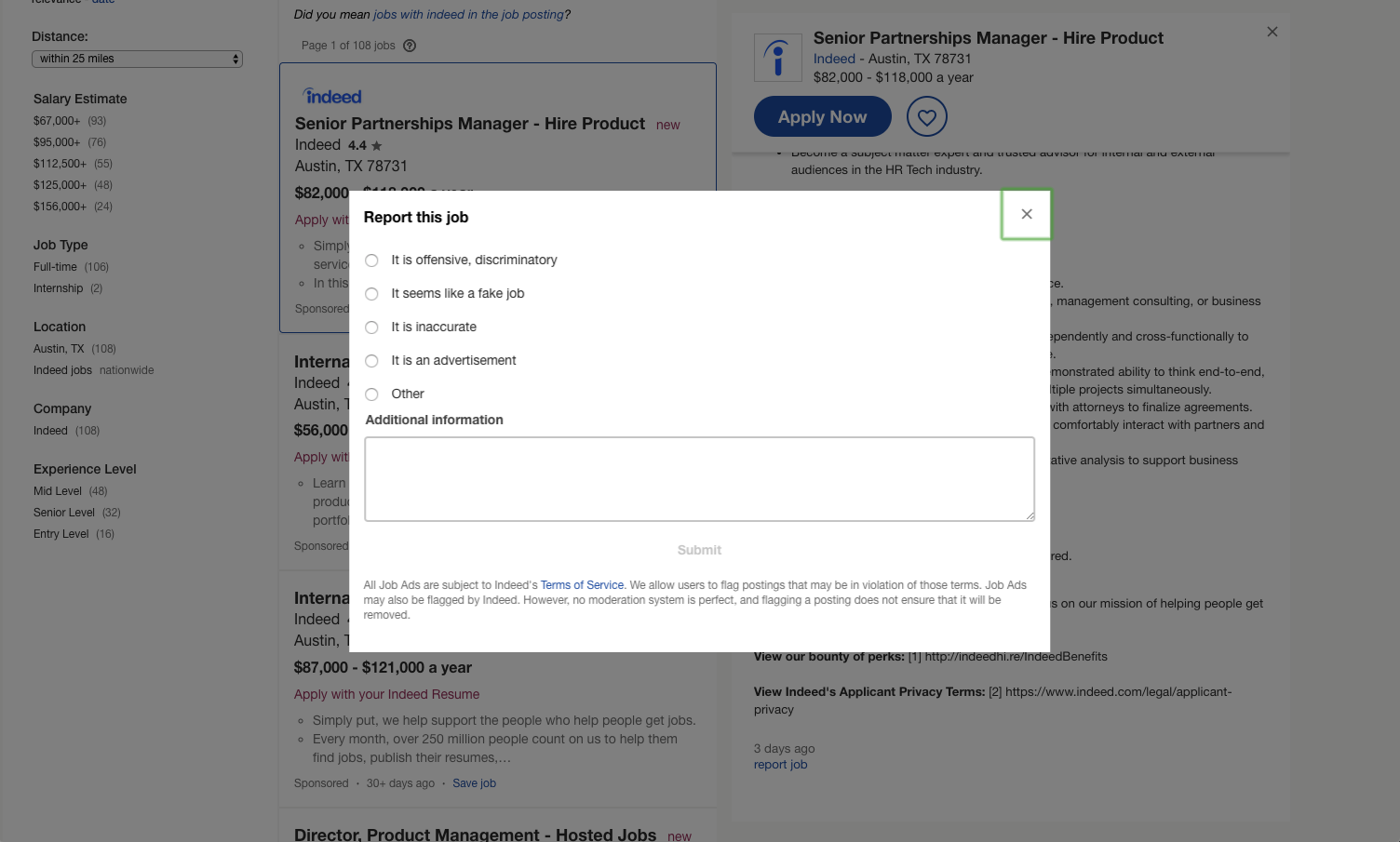Centered on the image is a white box labeled "Report this Job" at the upper left corner. Below the label are a series of selectable options presented as small circles, each with accompanying text. The options include "Offensive or Discriminatory," "Fake Job," "Inaccurate," "Advertisement," and "Other." Below these options, in black text, it reads "Additional Information," followed by a large, open text box for input.

The background is dimly shadowed, but key details emerge on the right side. The text reads "Senior Partnerships Manager – Higher Product," accompanied by a lowercase "i" inside a blue square. Next to this, the word "Indeed" appears in blue, along with the location "Austin, Texas, 78731" and the salary range "$82,000 - $118,000 a year." A blue circle on the right features the text "Apply Now," and a nearby circle contains a small heart icon.

To the left, the word "Indeed" reappears in blue, mirroring the job position information: "Senior Partnerships Manager – Higher Product," followed by the word "New" in red text.